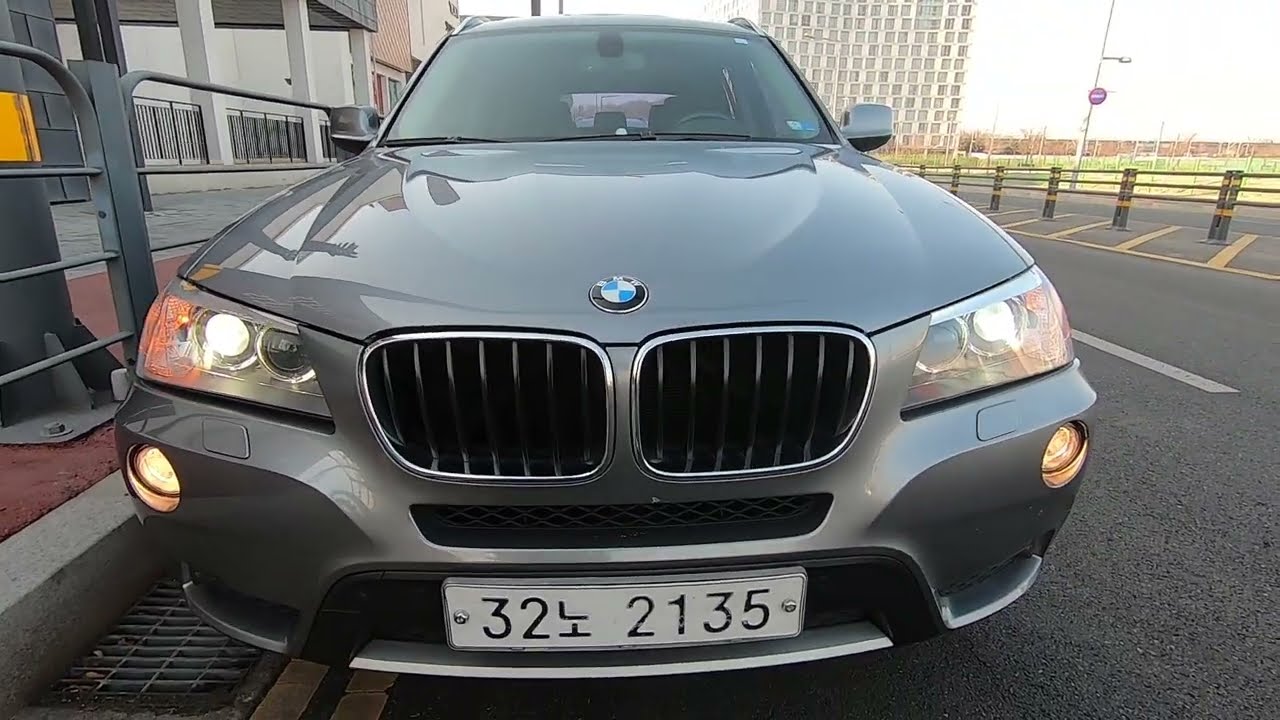The image showcases a light gray BMW car, prominently parked on a black asphalt surface during daylight hours, with its headlights switched on. The car’s front license plate, which reads "322135" with a symbol resembling an inverted 'T' or 'L' between the digits, indicates it is registered in a European country. The scene is set next to a sidewalk composed of red brick and separated by a light gray metal railing. To the right of the car lies a road marked by gray pillars with yellow lines. In the background, there's a building featuring white pillars, storefronts, and a multi-storied, cube-like residential structure. The sky overhead is light gray, while farther in the distance, a green grass field can be discerned. A distinct, circular red and white street sign is visible in the top right corner of the frame.